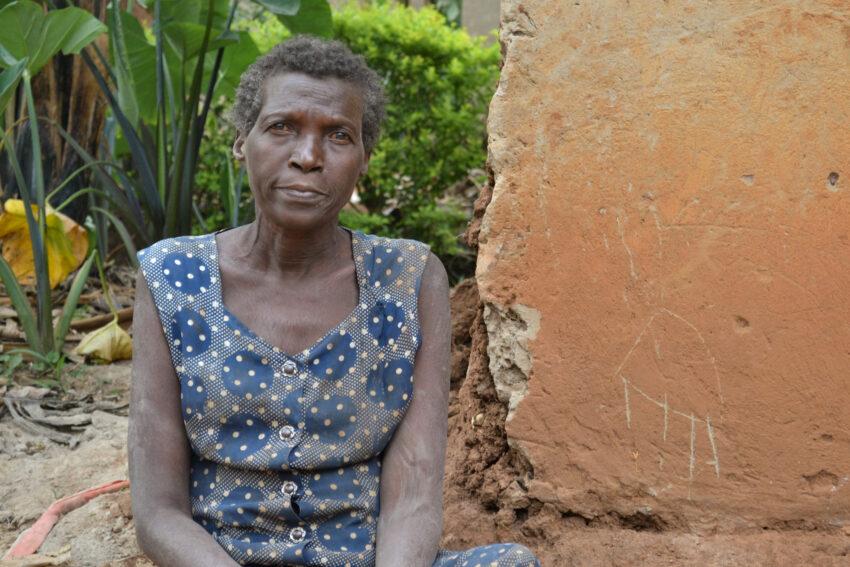The photograph captures a solemn, older woman with short, curly hair that is dark with hints of gray, and dark brown eyes, sitting on the ground next to a large rock. Her dark skin appears dirty, with a grayish tone, possibly due to a layer of clay. She is thin, with visible bones and clavicle, suggesting frailty. She is dressed in a sleeveless, button-up dress that is heavily soiled. The dress has a distinctive pattern featuring large navy blue circles interspersed with small white and yellow circles, and lines, with notably large metallic buttons.

The rock beside her, which is orange and beige in color, appears tall and stacked, adorned with carvings resembling an animal with a body and four legs. In the background, green foliage, yellowing leaves, and possibly the bark of a tree contribute to the natural setting. Despite her solemn appearance, there is a slight smile on her face, adding a poignant contrast to the scene's overall grimness.